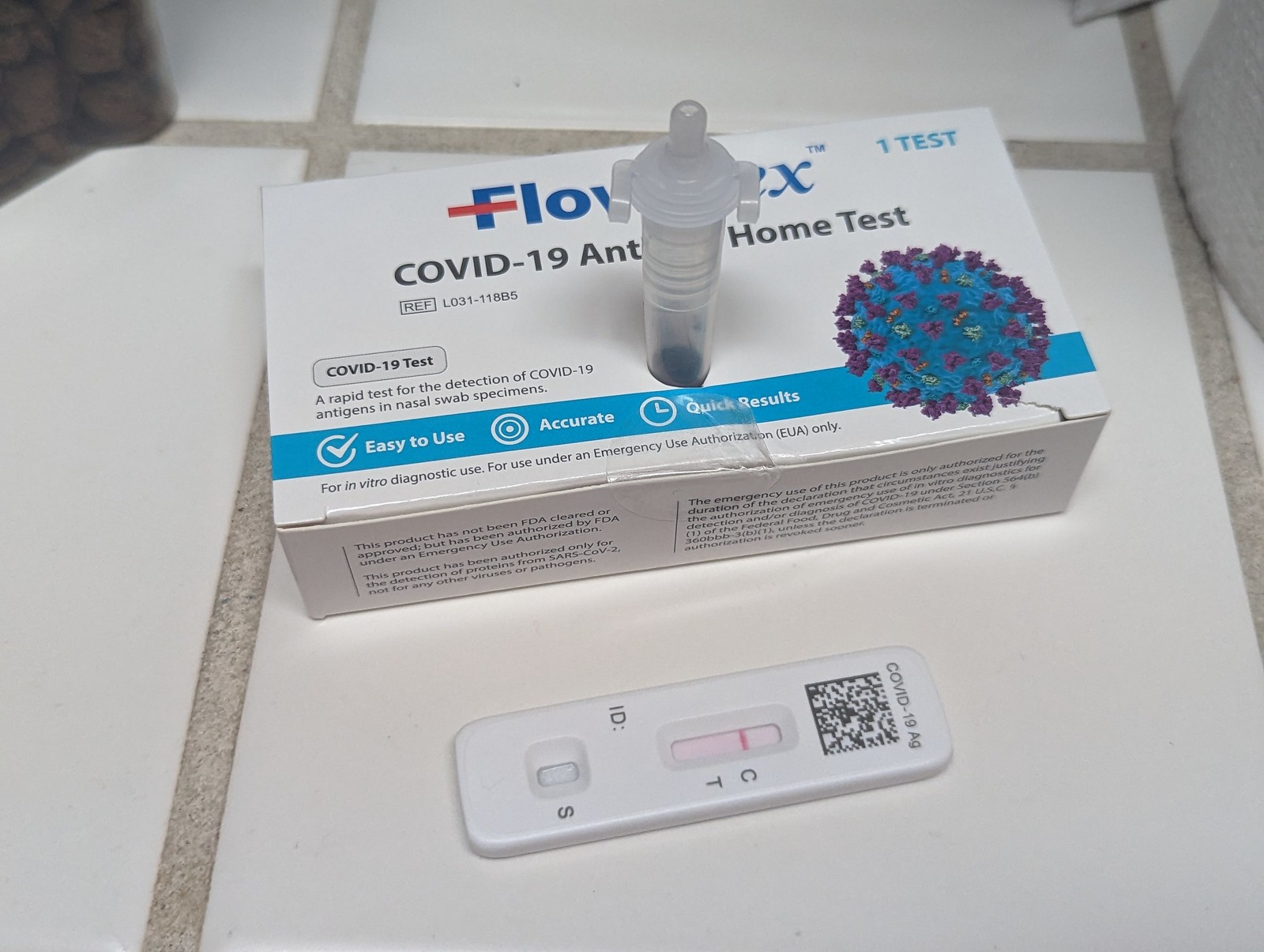On a white ceramic tile countertop, possibly in a kitchen or bathroom setting, sits a box of a COVID-19 home test. The pristine white tiles feature grout lines that enhance the clean, clinical look of the scene. The box prominently displays the partially obscured brand name "Flowflex," hidden behind a transparent tube projecting from a purpose-cut hole in the packaging. The text visible on the box reads "COVID-19 Antigen Home Test" and explicitly states that it is for "in vitro diagnostic use" and "for use under an Emergency Use Authorization (EUA) only."

On the right side of the box, an electron microscope image vividly depicts the coronavirus, showcasing its distinctive spike proteins (corona) that characterize the virus. Below the image, the box describes itself as "A rapid test for the detection of COVID-19 antigens using nasal swab specimens."

Accompanying the box on the tiles is a white plastic test device labeled "COVID-19 AG," which includes a barcode and features a small red stripe in an indentation aligned with the letter "C." At the bottom of this plastic component, the letter "S" is marked next to another indentation, crucial details for interpreting the test results.